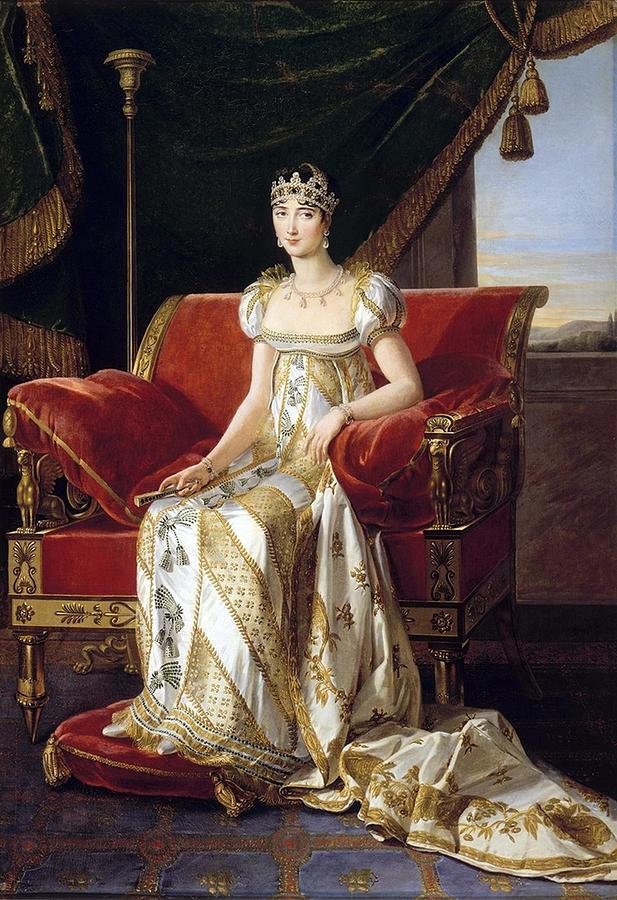This opulent painting depicts a regal woman—likely a queen or princess—seated on an ornate red velvet throne with luxuriant gold accents on its sides, armrests, and base. She is adorned in an elaborate white and gold gown featuring intricate patterns of flowers and leaves, and distinct diagonal stripes. The gown also showcases a prominent black pattern at its center. The sleeves are half-length and intricately designed, cascading down to the floor. 

The woman wears a diamond-studded crown with jewels, dangling diamond earrings, and a delicate diamond necklace, complemented by bracelets on her wrists. Her short hair and slightly tilted gaze add to her dignified aura. One hand rests on a red bolster pillow, while the other gently holds a stick or fan on her lap. 

Her feet are placed on a gold-trimmed red pillow taken from the throne, emphasizing her comfort and status. The background features a lush, dark green velvet drape with gold tassels and frills, partially revealing an open window. This window offers a glimpse of the sky and a portion of a hill, suggesting the painting is set within a grand palace. A nearby stand further enhances the scene’s grandeur, enveloping the viewer in an aura of royalty and luxury.